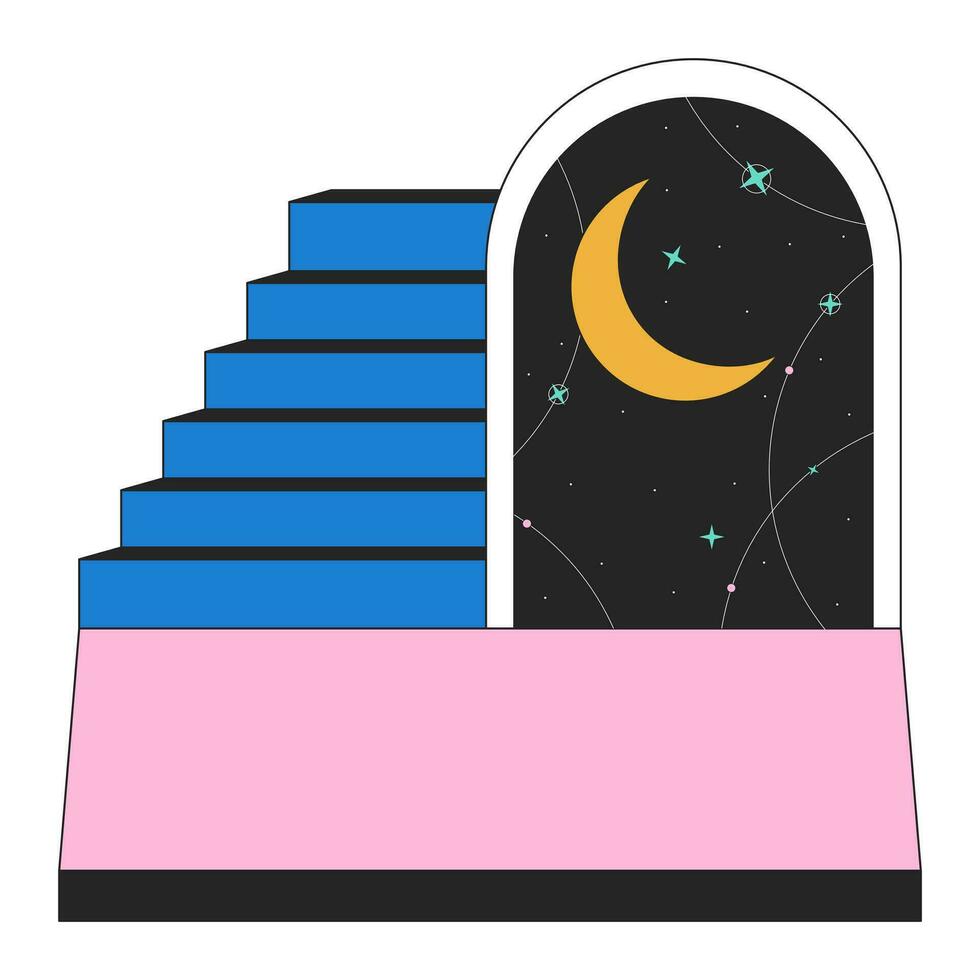The image is a detailed, colored drawing featuring a surreal and whimsical scene. At the bottom is a black border stretching across the entire width of the image. Directly above this black border is a thick pink rectangle, also running across the entire width of the picture. On the left side, a set of blue stairs consisting of six steps can be seen. These steps are widest at the bottom and narrow as they ascend. The top of each step is black, and the steps appear to lead nowhere as they are cut off by a tall pink wall behind them.

To the right of these blue steps, there is an arched window framed by a thin white border. This arch curves up from the top step, dips to the right, and descends down to meet the right edge of the pink rectangle. Inside this arched window, the background is black, adorned with twinkling blue stars and white lines that zigzag and curve, some encapsulating green stars. A yellow crescent moon is visible in the top left corner of this black space. Overall, the background of the entire image is white, providing a stark contrast to the vibrant colors and elements within the drawing.